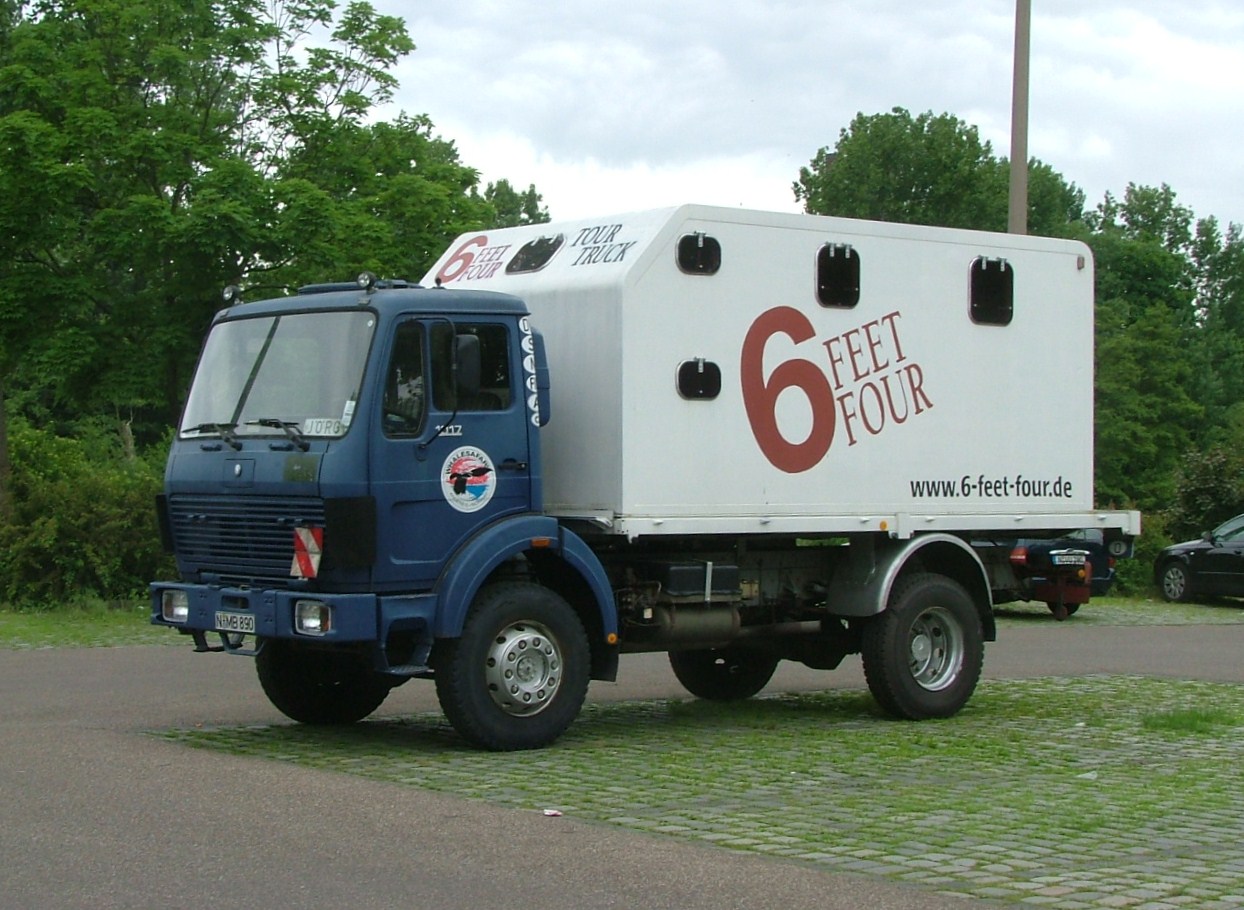The image is a landscape-oriented, real-life photograph taken outdoors, featuring a medium-sized truck facing sideways with its front pointing towards the left side of the frame. The truck has a distinct blue cab and a white trailer. Prominently displayed on the side of the trailer is large red text that reads "6 feet 4." Below this text, on the bottom right corner of the trailer, there is a website URL: "www.sixfeetfour.de." The truck is positioned on a grey tarmac surface and is equipped with four large black tires. In the background, there are green trees, a slightly cloudy sky, and two cars parked on the right-hand side, one of which is on concrete. Additionally, there is a pole, possibly a power pole, visible in the background. The area around the truck includes a section of brick with some grassy, weedy moss nearby. Overall, the image captures the truck as the central focus, with a natural outdoor setting providing context.